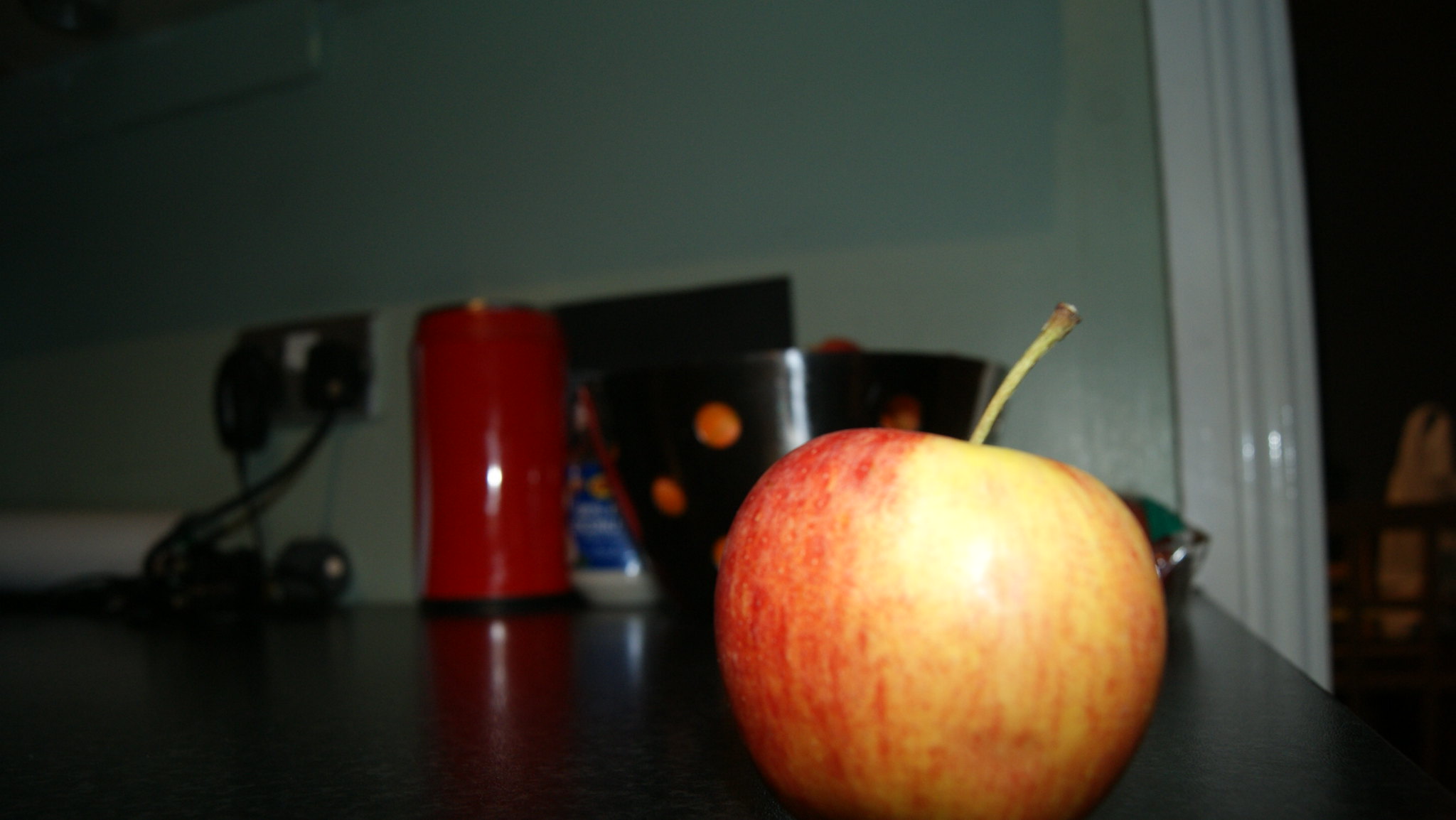The image depicts a cozy, well-used kitchen scene set within a house. Dominating the foreground is a glossy, reddish-yellow apple, showing more red on its sides and yellow towards its center, with light hitting it perfectly, causing a subtle shine. A small green and brown stem protrudes from the apple's top, adding a touch of detail. Positioned behind the apple, a black bowl with holes holds more fruit, possibly apples or other reddish-orange-colored produce.

To the left of the fruit bowl, there's a distinctive blue container adorned with a picture and some writing, adding a splash of color and character to the setting. Adjacent to that is a shiny red thermos, its metallic surface catching the ambient light.

In the background, a black angular object, possibly a monitor or the top of a chair, adds a hint of modernity contrasted by a white electrical outlet on the wall. The outlet has several black cables plugged into it, contributing to the kitchen's functional aspect. On the floor nearby, a white cylindrical object sits, its purpose unclear. 

The back wall of the kitchen is painted a soothing greenish hue, which gives the room a calm, cozy atmosphere. On the right side of the image is a white doorframe, through which a dimly lit area is seen, with faintly visible whitish elements in the darkened background, adding depth and mystery to the scene.